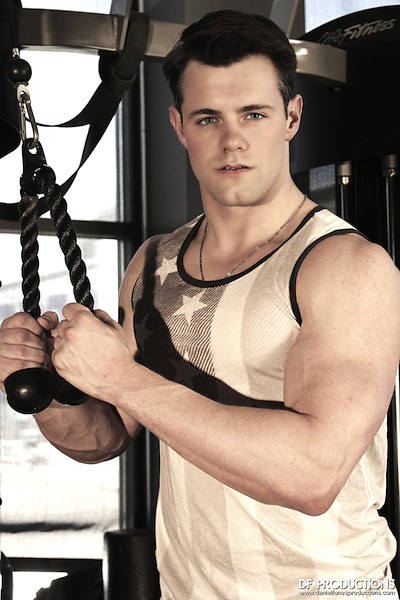The photograph features a muscular man in the midst of a workout, likely in a gym. Positioned on the right side of the image, he gazes forward, his slightly turned stance revealing short to medium-length brown hair. Dressed in a black tank top adorned with white stars on the right side and gray and white vertical stripes resembling the American flag, he appears focused and determined. His left arm is extended, gripping the ropes connected by a carabiner to an exercise machine, presumably for a triceps exercise. A silver necklace glints around his neck. In the background to the left, a window is visible, while the rest of the backdrop consists of a darkened gray wall. In the bottom right-hand corner, small text reads "DF Productions."